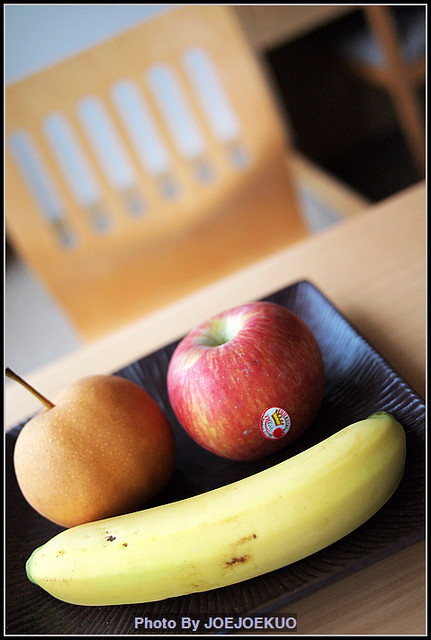The photograph features a small wooden bowl placed on a light brown wooden table, serving as the focal point of the image. The bowl is dark brown and contains three fruits: a red apple with a green interior, an orange apple with a small wooden stem, and a vibrant yellow banana with some black blemishes. A chair back can be observed in the blurred background, emphasizing the sharp focus on the fruit and bowl. Along the bottom of the image, the annotation "Photo by Joe Joe Kuo" is rendered in white font, contributing to a serene and homely composition.